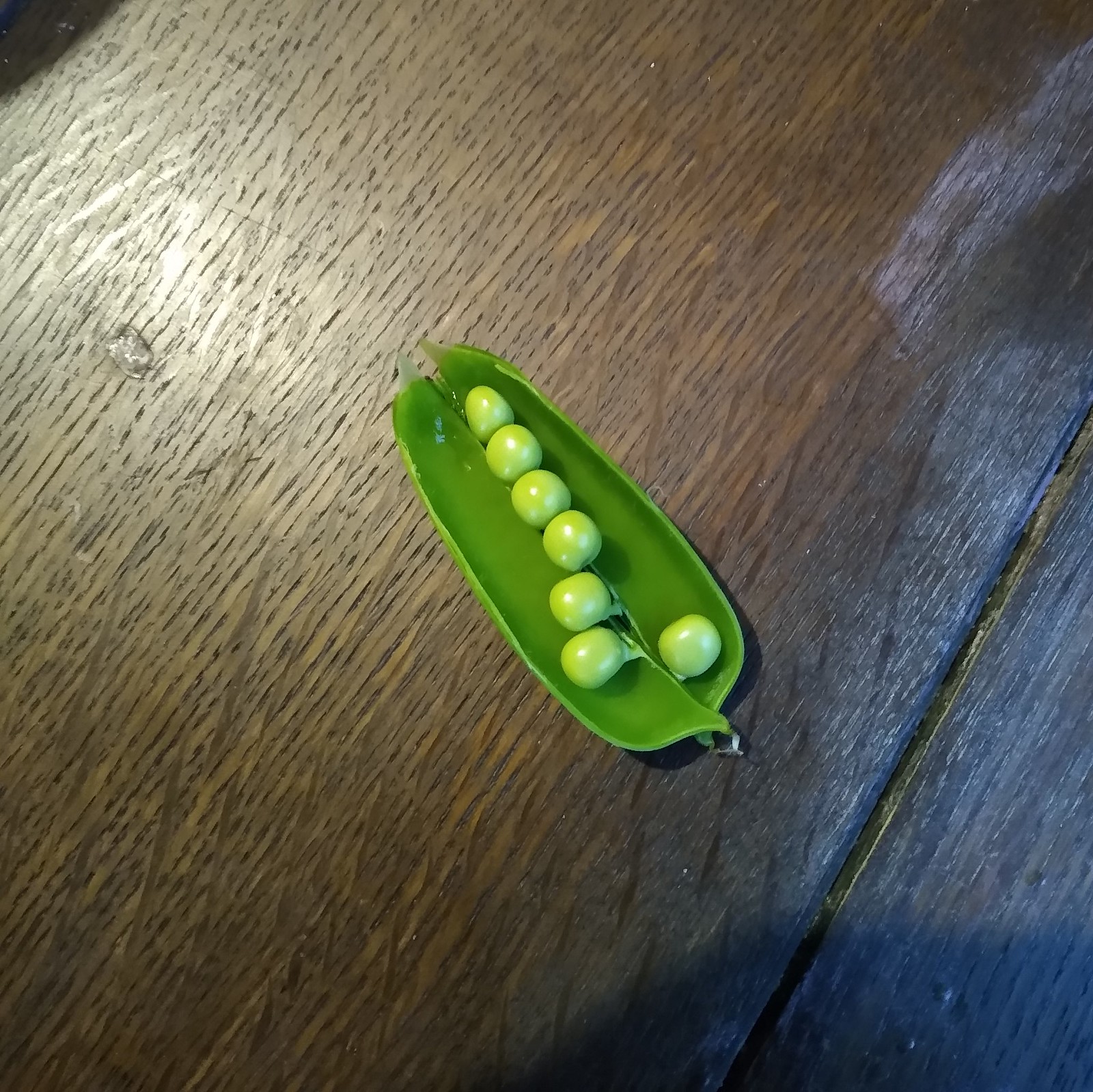In this color indoor photograph, the subject is an opened, plastic peapod containing seven plastic peas. The peapod exhibits a dark green hue, while the peas are a light green color, enhancing the contrast between them. It's placed on a brown, wooden surface with distinct wood grain patterns. The table or desk, perhaps made of oak, shows a subtle seam between two planks, and there's a noticeable water stain in the lower right corner, casting a shadow that darkens that area. Light enters from the upper left corner, illuminating that part of the surface. The peas are arranged with six clustered towards the left and one separated on the right, giving a detailed, textured depiction of both the peapod and the wooden tabletop.